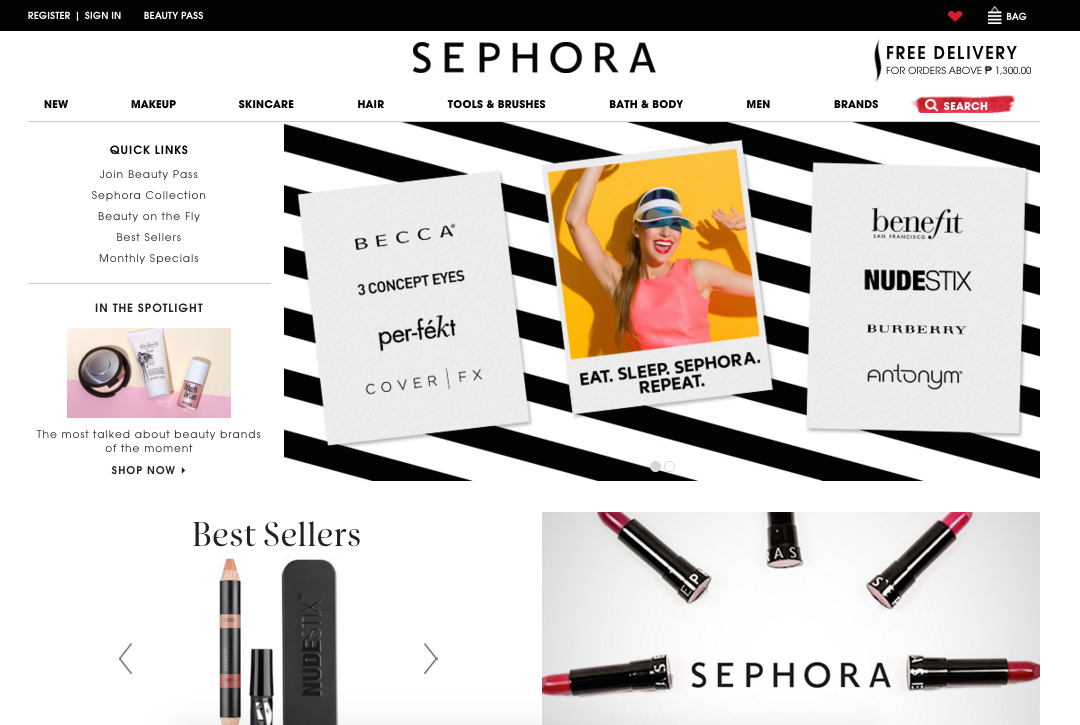This screenshot captures the main page of Sephora's website, presenting a comprehensive view of its interface and key features.

**Header Section:**
- **Top Left Corner:** Displays options to "Register," "Sign In," and access the "Beauty Pass" program.
- **Top Right Corner:** Features a shaded red heart icon next to the "Bag" icon, which is depicted with horizontal lines.

**Main Page Content:**
- **Sephora Logo and Offer Banner:** The Sephora logo is prominently displayed at the top, against a white background. Below it, a banner announces "Free Delivery for Orders Above ₱1300," indicating currency tailored possibly for the Philippines (₱ for Philippine peso).
- **Navigation Tabs:** Just beneath the banner, there are navigation tabs for various categories— "New," "Makeup," "Skincare," "Hair," "Tools & Brushes," "Bath & Body," "Men," and "Brands." Notably, "Bath & Body" uses an ampersand for "and."

**Search Bar and Quick Links:**
- **Search Bar:** Highlighted in red, featuring a unique crayon-style font, inviting users to type in their queries.
- **Quick Links:** Located under the navigation tabs, showing options like "Beauty Pass," "Sephora Collection," "Beauty on the Fly," "Bestsellers," and "Monthly Specials" in lighter gray text.

**Right Column and Visual Elements:**
- **Slideshow Images:** The right column features three sections with different visuals. The active and inactive statuses of the slideshow images are indicated by circles— one grayed out and another open.
- **Promotional Image:** One of the key images states "Eat, Sleep, Sephora, Repeat." A woman in the visual, with a blue visor, red lipstick, and pink top, has her hair in a long ponytail extending past her armpit. She poses energetically with both hands raised.
- **Additional Graphics:** Accompanying the woman are various makeup items, including prominently displayed red lipstick and other beauty products.

This detailed description encapsulates the essence of the Sephora main page, from the header contents to the promotional visuals and navigation aids—a comprehensive guide for what a user might see when they first visit Sephora's website.